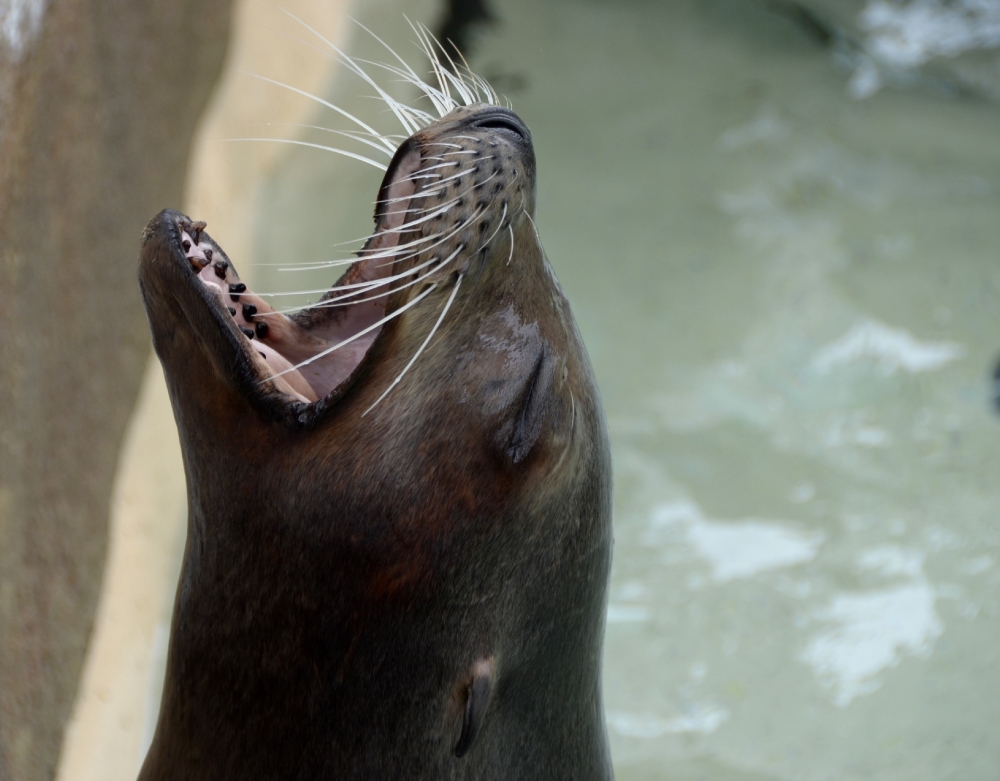The image is a close-up of a brown seal’s head, depicted in a rectangular, almost square, horizontal frame. The seal's eyes are shut, and its mouth is wide open, revealing a pinkish tongue and small black and dark yellow teeth. Prominent white whiskers frame its face, which is predominantly black. The seal's one visible ear is located in the bottom middle of the image. The background is blurred but shows a body of churning, light greenish water, suggesting the seal is near the edge of an enclosure or pool. The shot captures the seal from the neck up, focusing on intricate details like the inside of its mouth and its facial features, giving the impression that the seal might be awaiting food.